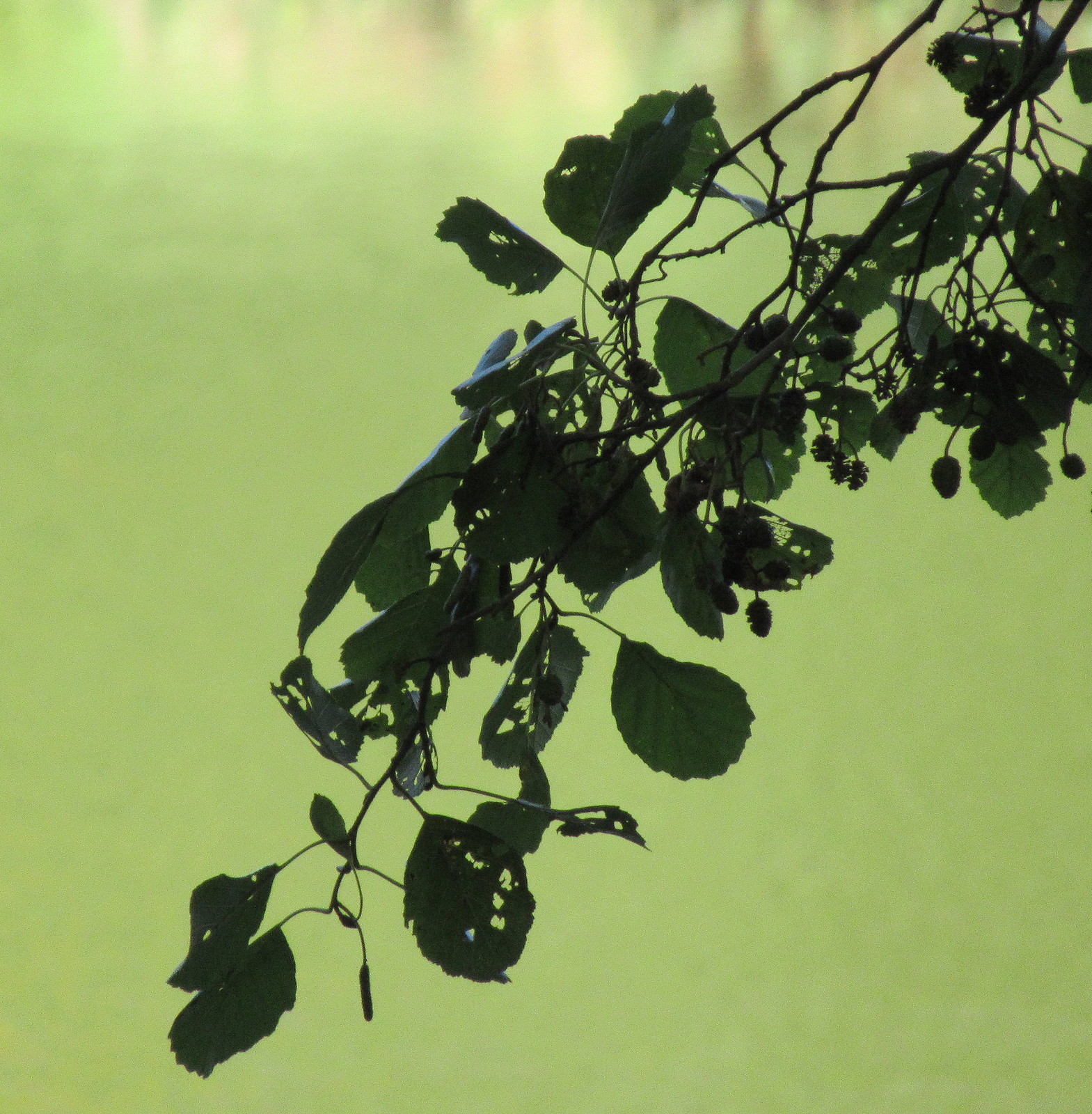In the image, a delicate, spider-like branch extends from the upper right corner, adorned with numerous round or lobed green leaves, some of which are eaten away, revealing small holes through which light passes. Among the leaves, you can spot tiny catkins hanging. The leaves and branches, possibly from an alder tree, span across the frame, with the foliage ending in the bottom left corner with two prominent leaves. The background is a gradient of lime green, transitioning to a more yellow hue towards the top left, possibly hinting at a reflection on green water or a yellow-tinted sky. The overall scene creates a serene and detailed depiction of a natural, outdoor setting.